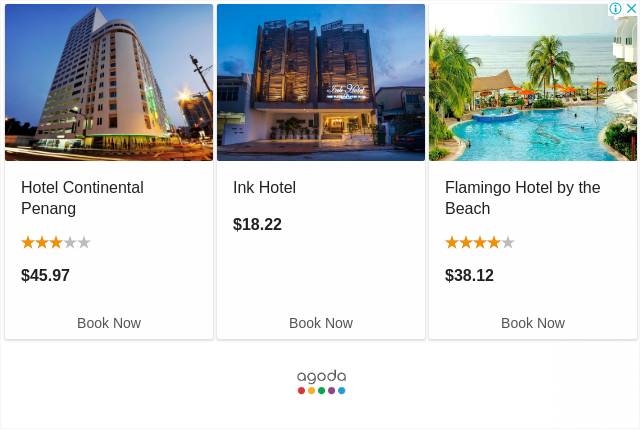This image showcases three different hotels, each presented with booking details. On the left, we have Hotel Continental Penang, rated three out of five stars, with a price listed as $45.97. A "Book Now" button is prominently displayed at the bottom in gray font. In the middle, there's Inc Hotel, priced at $18.22, also accompanied by a "Book Now" button. Finally, on the far right, Flamingo Hotel by the Beach is featured, boasting a four-star rating and a price of $38.12, with a clickable "Book Now" option. At the very bottom center of the image, the word "Agoda" is present, underscored by five colored circles: red, yellow, green, purple, and teal.